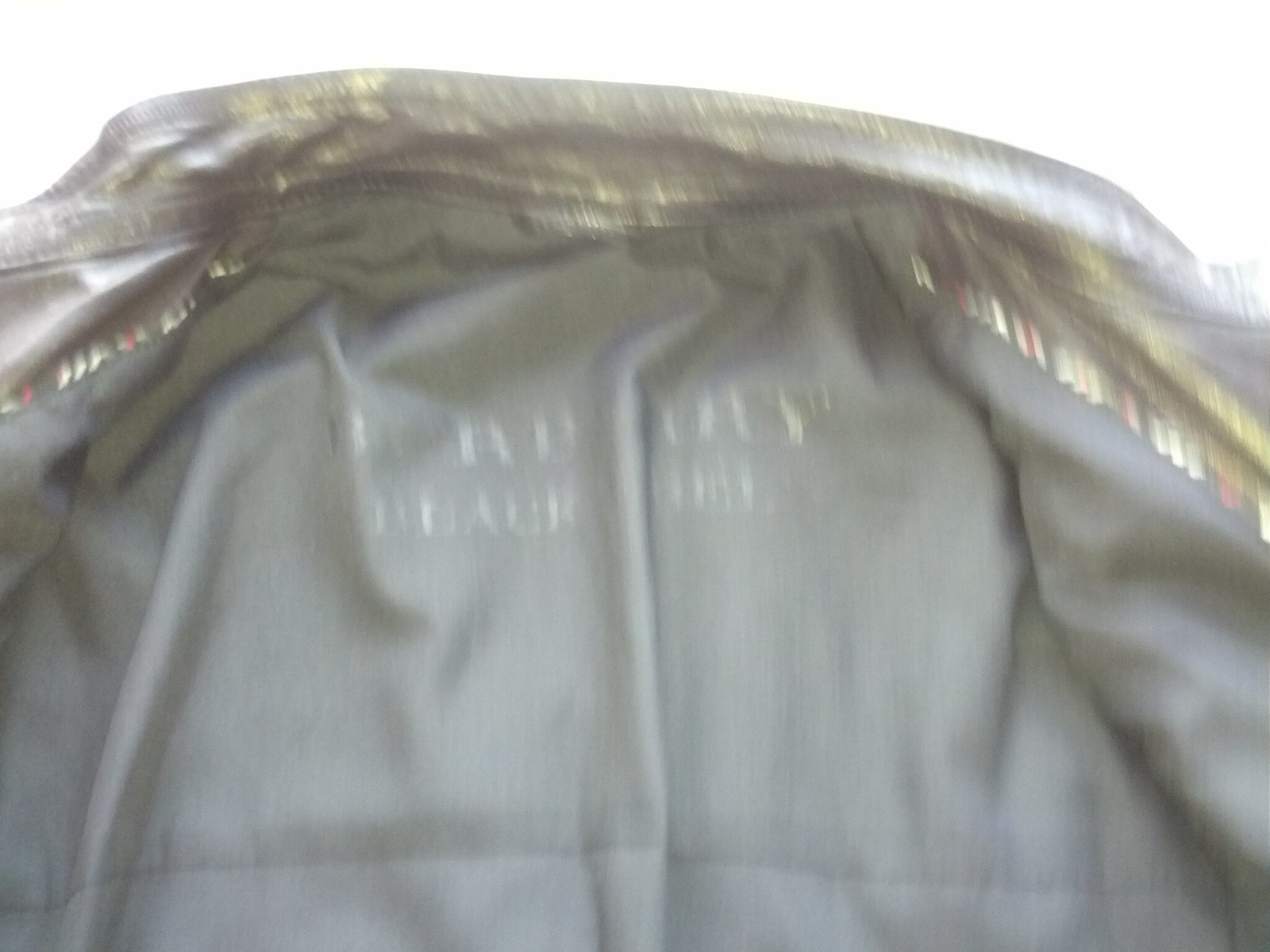This is a color photograph depicting a close-up view of the interior of a jacket, though it's quite blurred, making the finer details indistinguishable. The jacket appears to be a greyish-green hue. The background is predominantly white, providing a stark contrast to the jacket's color. The focus is on the area just below the collar, where a logo is printed inside the jacket. Although the lettering is white and spans two lines, it's too blurry to discern the text. The fabric exhibits some creasing at the center, causing a separation between the lines of text. 

The collar itself is visible, decorated with stripes in a combination of light white, yellow, red, and possibly black. The very top of the neckline showcases a mottled black and yellow pattern. There's a seam running down the middle of the jacket, further suggesting its construction as a rain jacket. Despite the blur, the image offers an intimate view of the jacket’s inside features and details, which may be useful for someone familiar with this specific brand or style.